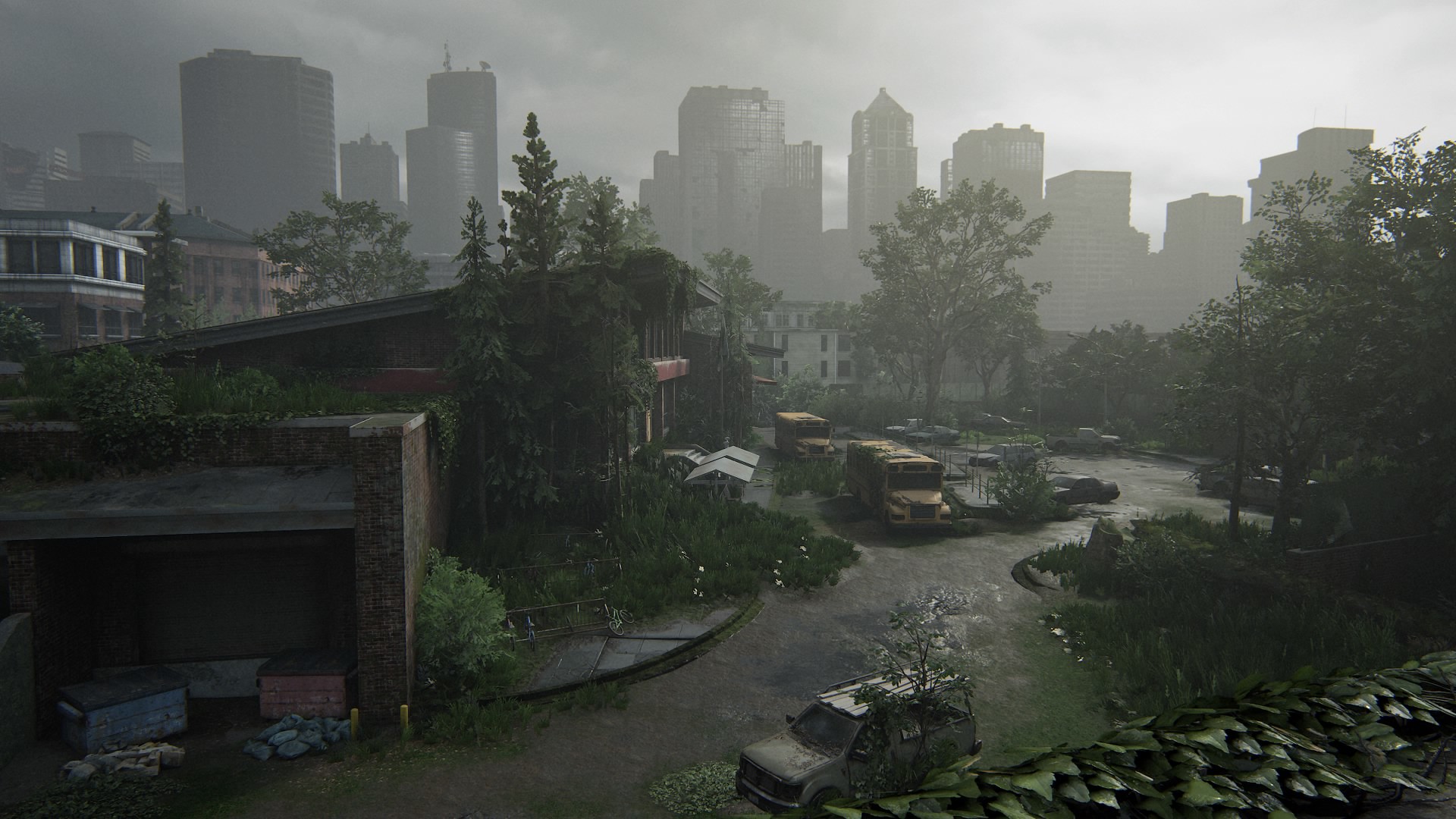A haunting image of a deserted town is portrayed, where the encroachment of nature is vividly apparent. At the forefront, a car partially engulfed by a robust tree illustrates the passage of time and neglect. In the background, a collection of vehicles, including a couple of buses and an array of other cars, sit parked in disarray, seemingly forgotten. Nature’s claim is evident with colossal vines and dark green leaves spreading out from the far right-hand corner, creeping over the lifeless vehicles. The town’s sense of abandonment is further emphasized by the many buildings standing vacant and desolate under an ominous dark gray sky, shrouded by overgrowing trees, vines, and dense foliage.